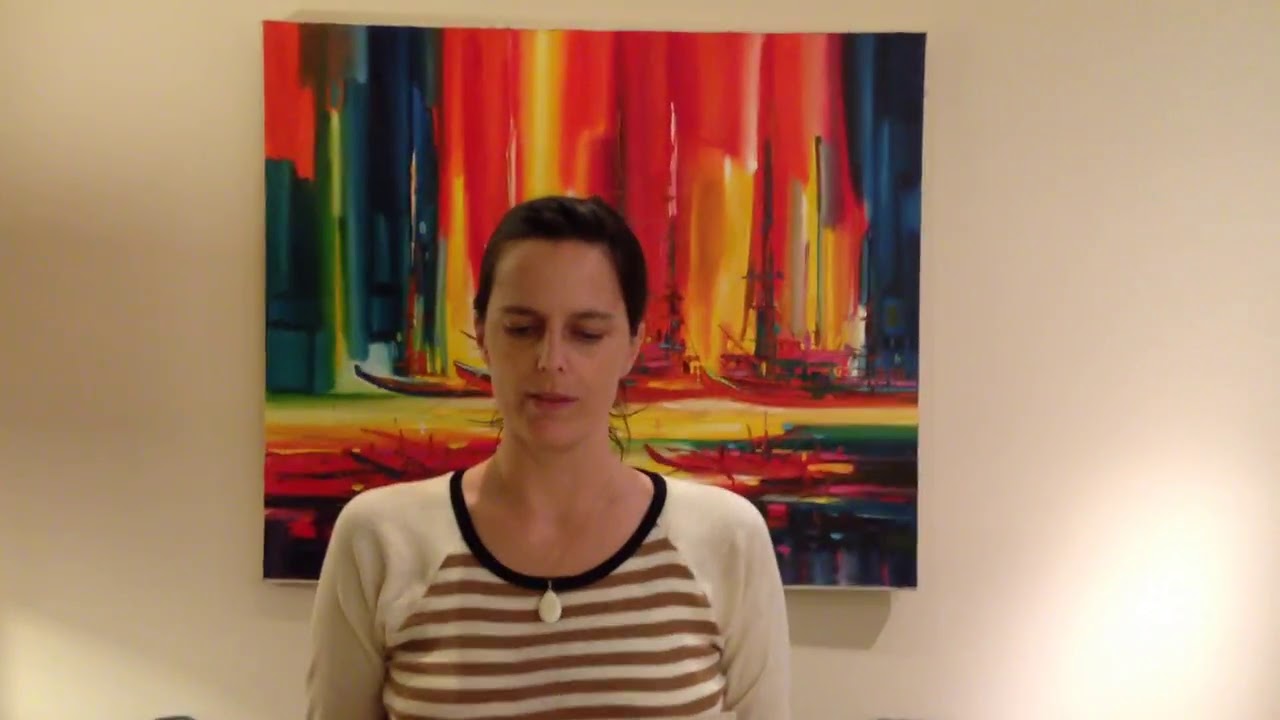This is a photograph of a young Caucasian woman, likely in her late teens or early 20s. She has dark brown hair pulled back into a ponytail with a few wisps framing her face. She has an oval face with dark brown eyebrows and long dark lashes, and her eyes are closed or cast downward, giving her a contemplative or relaxed appearance. The woman is wearing a beige sweater with a black outline around a rounded neckline. The center of the sweater features horizontal stripes in white and tan, and it has raglan-style sleeves. Draped around her neck is a gold necklace with a pendant, resting just above her chest.

The background of the image shows a room with a beige wall, adorned by a brightly colored painting. The painting is highly vibrant, featuring vertical and horizontal lines in a rainbow of colors including red, blue, yellow, green, orange, and deep cobalt blue. The colors blend and ripple across what might be cellophane-like elements or a textured surface that forms part of the painting. No other people are present in the photograph, and the woman's position captures her from mid-torso to the top of her head, suggesting she could be engaged in thought or possibly speaking mid-sentence in a video.